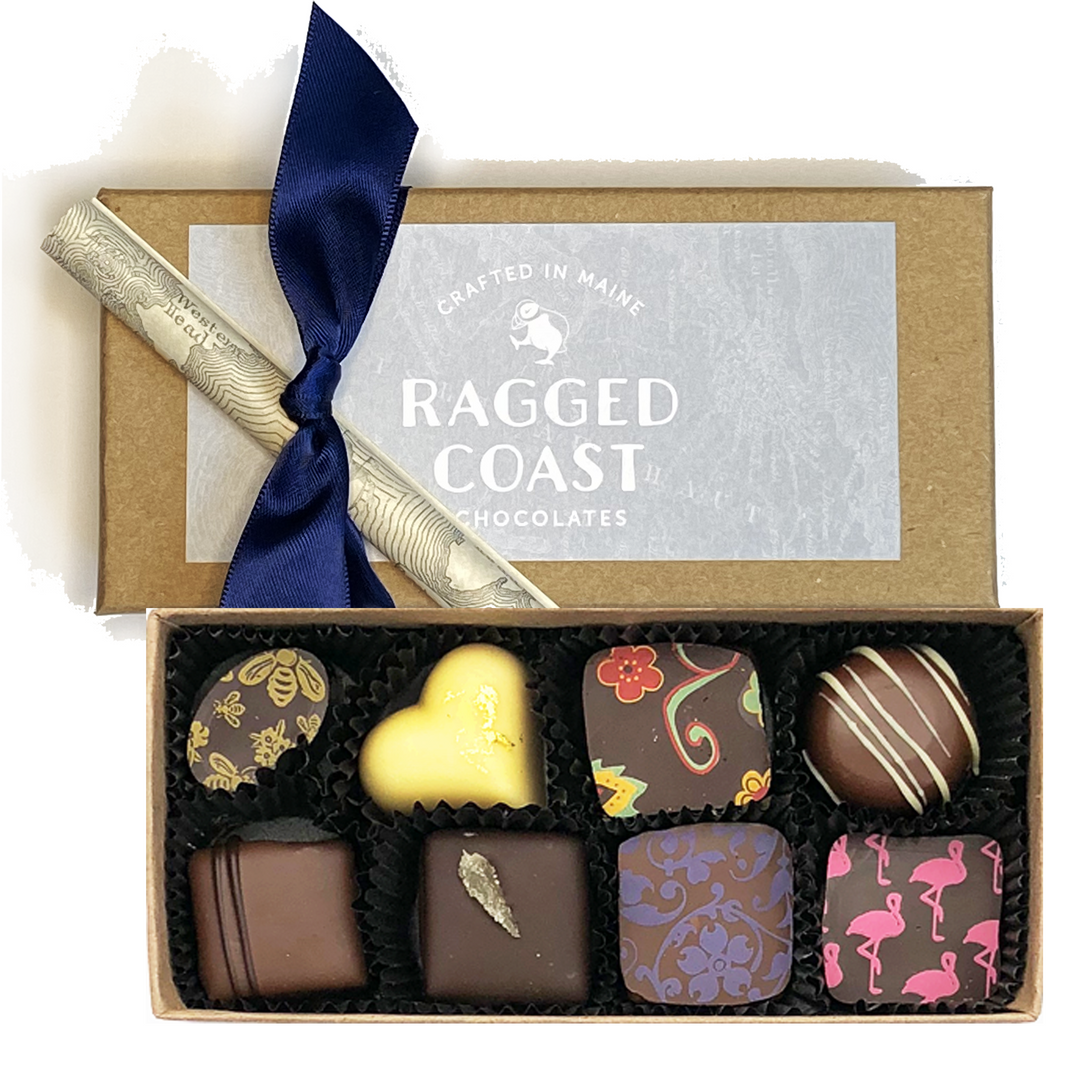This image showcases a beautifully crafted box of artisanal chocolates. The box, made from natural craft brown paper, has its lid placed face up, prominently displaying a light gray label that reads, "Crafted in Maine, Ragged Coast Chocolates." Below the box is a rolled piece of paper resembling a map, tied with a dark blue satin bow.

Inside the box, there are eight exquisite chocolates nestled in little brown paper cups. The assortment includes five square chocolates, an oval chocolate, a round chocolate, and a heart-shaped chocolate. The heart-shaped piece stands out with its gold hue. The oval chocolate features a distinctive bee pattern, while the round chocolate is adorned with white striping on a brown base. The square chocolates are decorated with various intricate designs: one has pink flamingos, another is embellished with a blue floral pattern, one has a tiny gold leaf, another features colorful striping over a red flower, and the last square chocolate has two dark chocolate lines on the left side.

This detailed presentation highlights the craftsmanship and artistry poured into each piece of chocolate, making it a true visual and culinary delight.